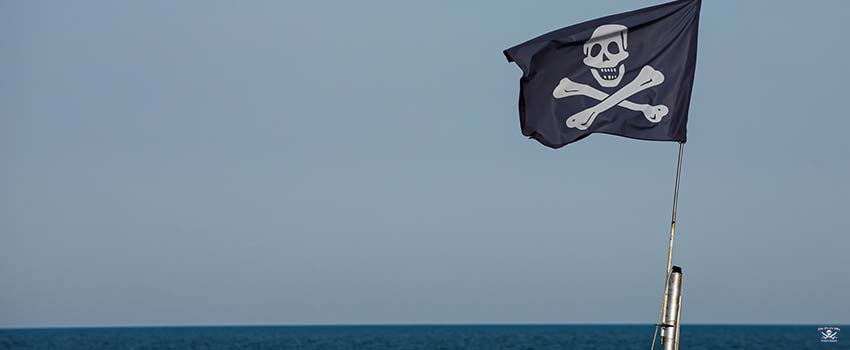A striking image centers on a black Jolly Roger flag waving from a silver pole against a vast blue, cloudless sky. The iconic pirate flag features a white smiling skull above two crossed femur bones. The background is dominated by the light blue sky, which occupies most of the frame, making up approximately seven-eighths of the image. Below this expansive sky, a thin strip of dark blue ocean stretches along the bottom. On the lower right-hand corner, a small white logo is visible, though the accompanying text is too small to read. The logo seems to depict another skull with crossed lines, adding to the maritime theme. The flag, likely mounted on a ship's mast, ripples gently in the wind, embodying a classic pirate motif.